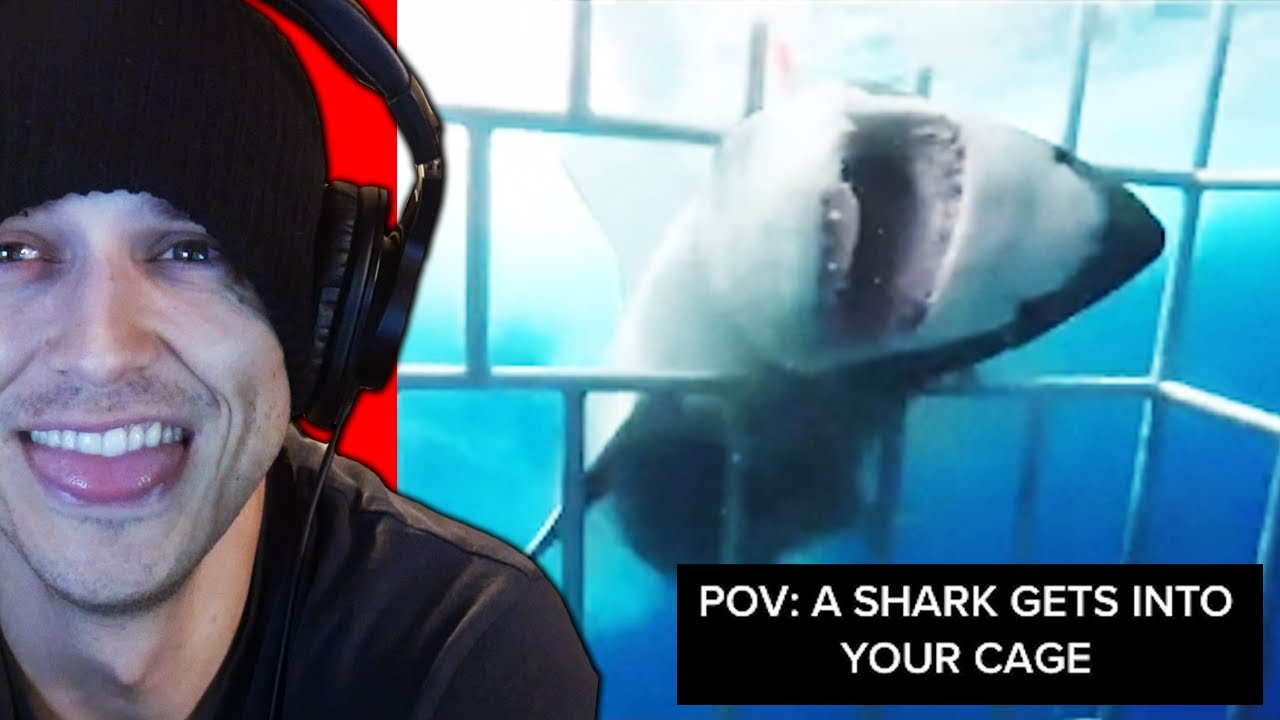The photograph captures a unique juxtaposition of two primary elements within a split-screen format. On the left side, a young Caucasian man, donned in a black hat, black shirt, and black earphones, is beaming into the camera with a charismatic smile, even sticking his tongue out slightly, indicative of a cheerful, possibly humorous mood. He appears to be engaged in a podcast or show, seated indoors with a casual and relaxed posture. To the right, the scene shifts dramatically to an underwater setting, saturated in various shades of ocean blue. Here, a shark, characterized by its gray and white coloration with a notably open pink mouth, has its head stuck through the bars of a cage, angled slightly to the east. In the bottom right corner of this aquatic scene, white text reads “POV: A shark gets into your cage,” capturing a vivid moment of underwater tension. The colors in the image range from dark ocean blue to light ocean blue, white, gray, black, red, and beige, adding depth and contrast to the visual experience. The entirety of the image conveys a stark, almost surreal blend of human lightheartedness and the wild unpredictability of marine life.